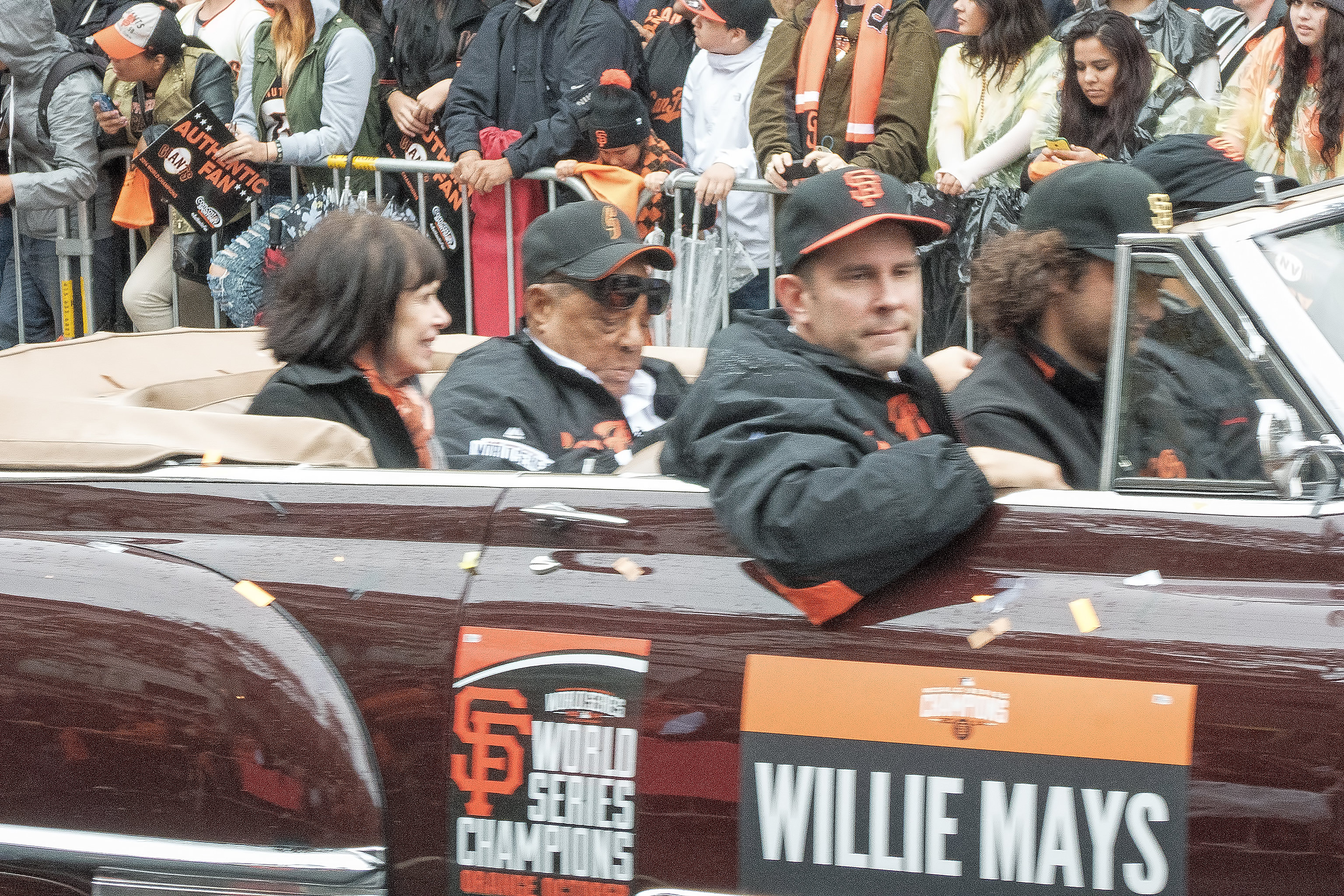This photograph captures a festive baseball parade celebrating the San Francisco Giants' World Series Championship. Central to the image is a classic, burgundy-colored convertible with Willie Mays seated in the back, accompanied by a woman. Mays, wearing a black and orange San Francisco Giants cap and matching jacket over a white shirt, is seen with his sunglasses slightly lowered, revealing his eyes as he looks down. The car prominently displays a sign reading "Willie Mays" along with another sign mentioning the San Francisco World Series Champions. In the front seat, three younger baseball players are dressed in San Francisco Giants uniforms, caps, and jackets. One player is casually resting his arm on the passenger side of the car. Behind the convertible, a lively crowd of spectators, penned in by a white rail fence, holds signs and cheers, adding to the celebratory atmosphere. The scene encapsulates a moment of honor for Willie Mays, amidst the joyous celebration of the Giants' victory.